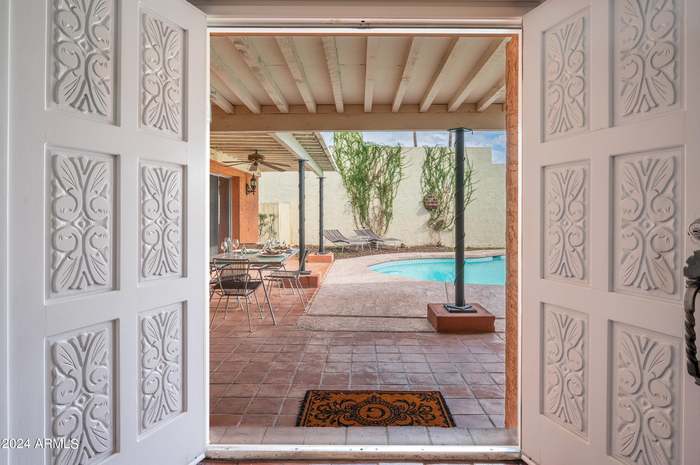A serene outdoor setting featuring two elegant, pale gray double doors adorned with intricate floral and leaf carvings. In front of the doors, a brown doormat with a floral design centers around a prominent letter 'G'. The area boasts a tile floor that surrounds a sizable blue pool. Encircling the space is a tall concrete wall, partially draped in lush green vines, adding to the tranquil atmosphere. A spacious patio area provides ample seating with various tables and chairs, all sheltered under a canopy, inviting guests to sit back and unwind in this peaceful haven.